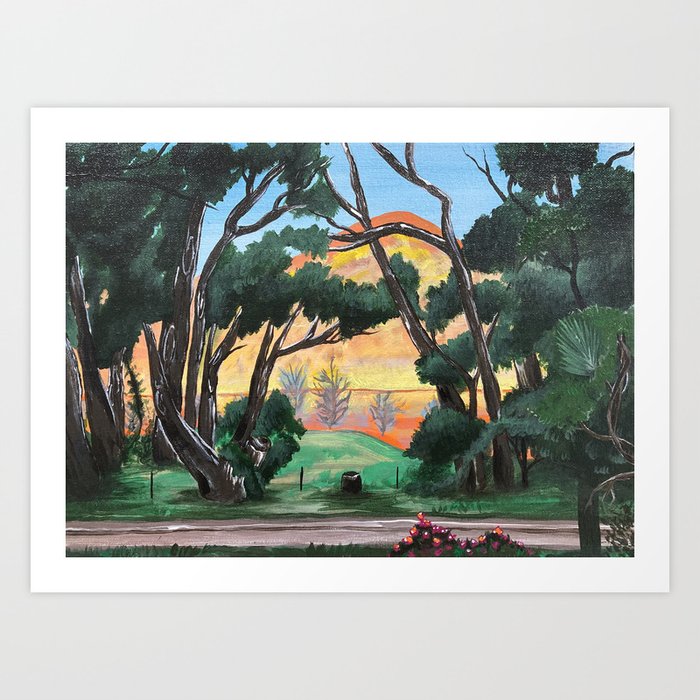This painting, rendered in a realistic, photographic representationalism style by Lisa Lindsay, beautifully captures a tranquil daytime outdoor landscape set in the Australian bushland near Lake Eldon. Dominated by tall trees with bending trunks and lush green leaves, the detailed artwork presents a forest scene with a dirt road cutting through the middle ground. The foreground features a gray stream accompanied by pink flowering shrubs and vibrant green grass, adding a burst of color against the natural backdrop. In the background, a majestic mountain, with striking red and gold hues reminiscent of a pyramid shape, rises grandly, partially obscured by trees standing on sandy soil. Nestled behind these trees is a yellow-orange house with a red roof, its gable peeking through the canopy under a vast blue sky, creating a juxtaposition of natural beauty and subtle human presence. The painting is framed with a white border, all set against a light gray background.